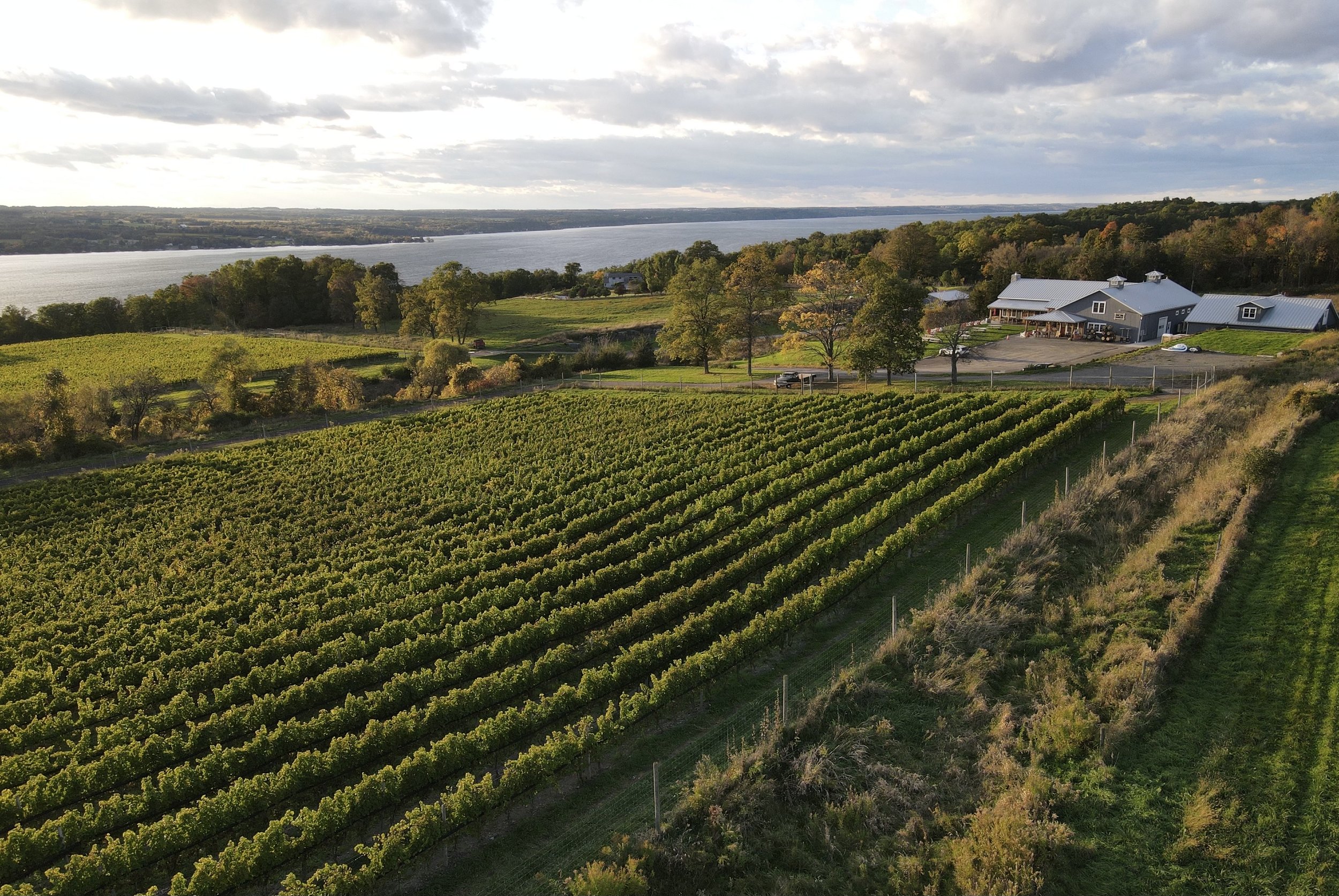This color photo captures a serene countryside landscape under a light gray sky dotted with clouds. The lower part of the image is dominated by meticulously cultivated rows of green crops, stretching diagonally from the bottom left to the upper middle of the image. To the right of these rows, a dirt path flanks a white-posted fence that runs up to the middle of the image, marking the boundary between the cultivated area and a more unkempt grassy region dotted with small bushes.

In the upper right corner, there's a cluster of buildings that look like houses or barns, partially obscured by tall trees behind them. Toward the left, there's more greenery—a mix of grassy areas, bushes, and trees lining a riverbank. The river flows from the upper left, snaking its way behind the trees and extending towards the horizon. The upper portion of the image features the sky, occupying about a fifth of the frame and lightened by a mix of white and light blue clouds. In the distance, beyond the trees and buildings, stretches a bluish land, adding to the tranquility of the pastoral scene.